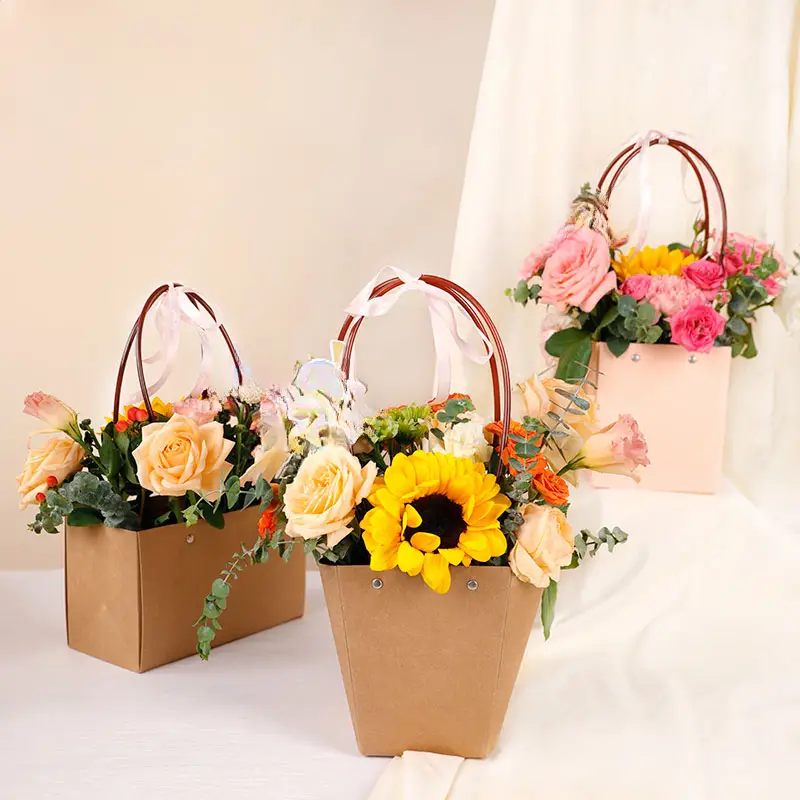The studio photograph captures a vibrant and colorful arrangement of three bags filled with various flowers, set against a flowing white curtain backdrop. In the foreground is a U-shaped, light brown tote bag adorned with a light pink ribbon on its pink handle. This bag hosts a diverse assortment of flowers, including sunflowers, light yellow and pink roses, an orange bloom, and assorted greenery. Positioned behind this tote to the left is a similarly shaped light brown bag, also featuring a pink ribbon on its handle. This second bag contains a mix of pink roses, tulips, and lilies. The third bag, located at the back on the right side, stands taller and is light pink with a square shape. It includes a handle with a pink ribbon, similar to the others, and is filled with pink roses, various pink flowers, and sunflowers. The bags, made from a box-like, riveted cardboard material, showcase meticulous rivet details in the front, adding an element of craftsmanship to the display. All bags are semi-centered within the frame, creating a balanced yet dynamic presentation of floral beauty.